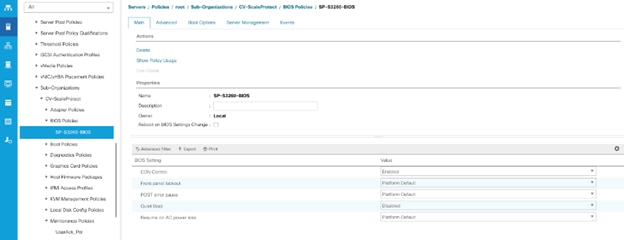The image appears to be a screenshot of a computer page with several distinct sections. On the left, there is a vertical blue banner featuring various icons, though the icons are difficult to discern due to their small and somewhat blurry appearance. To the right of the blue banner is a white rectangular area with a search bar at the top. Below the search bar, there are several bullet points listing items in black text. This section includes a blue-highlighted area in its middle portion.

To the right of this vertical area, a larger section dominates the page. At the top of this section, there are seven horizontal tabs—six are blue and the seventh is black. Below these tabs, there are five clickable blue tabs with blue text. Further down, the section contains multiple lines of phrases or words, stacked vertically. Despite the detailed structure, the text throughout the entire image remains small and blurry, rendering it unreadable.